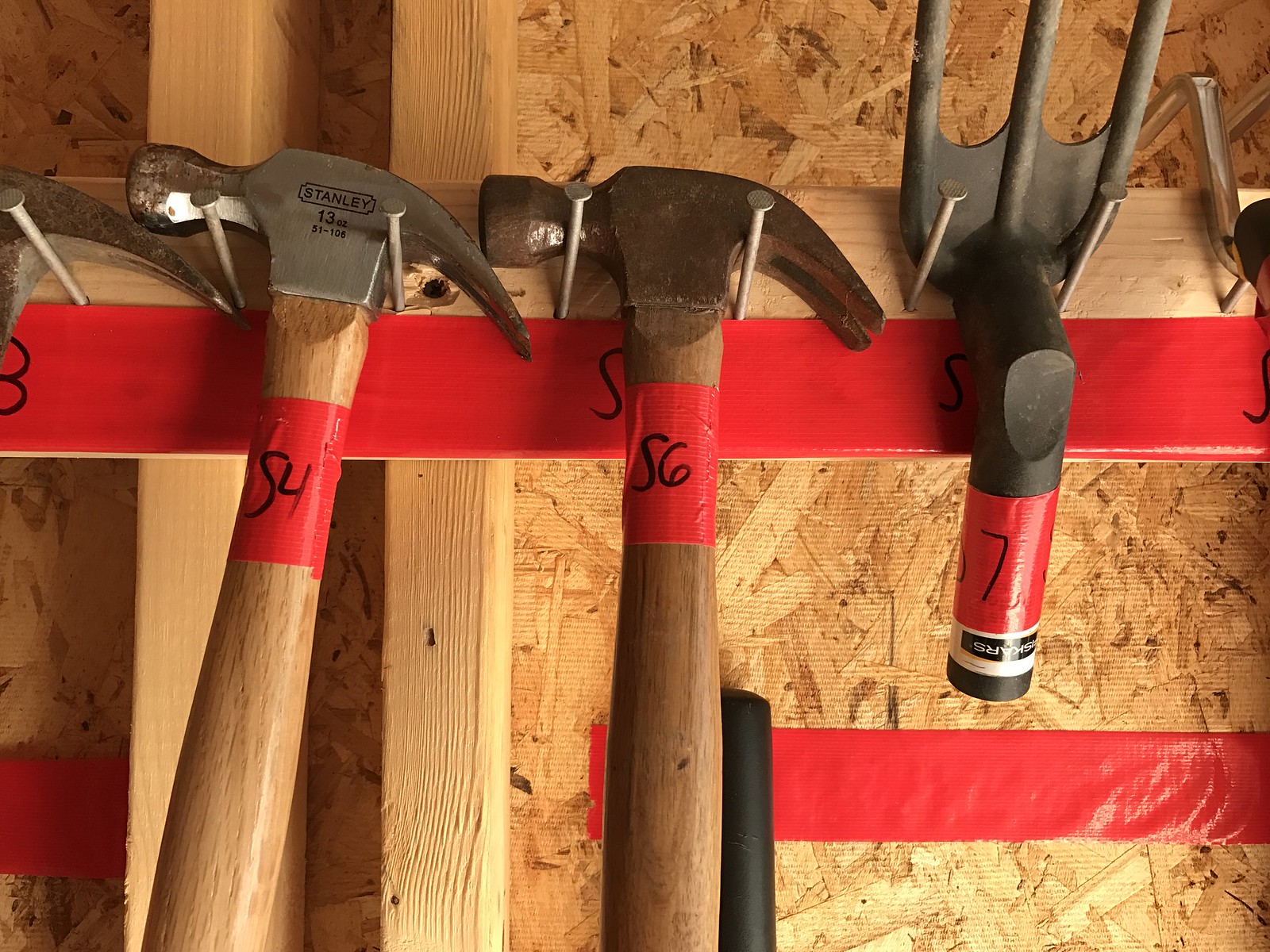The photograph captures a detailed scene within a shed, where a variety of tools are neatly organized. Dominating the upper portion of the image is a horizontal 2x4 plank, which is affixed to a brown flake board wall. Attached to this plank with three-to-four-inch flat-headed nails are two claw hammers and a garden hand rake. The hammer to the left, identified by its silver head and black-lettered "Stanley" logo, bears the marking "S4" in black pen. The central hammer, older with a rusted head, is marked "S6." Both hammers' heads are oriented to the left. To the right of these hammers is a black-handled garden rake with three prongs, also marked with the number "7" in black pen. All tools feature red tape around their handles, corresponding with the numbers inscribed on them, ensuring easy identification and organization.

Additionally, another strip of red tape is seen horizontally across the lower half of the 2x4 and in the lower right corner of the image, providing a visual guide for tool placement. The overall scene suggests a well-maintained, methodically organized workspace within the confines of a wooden shed.